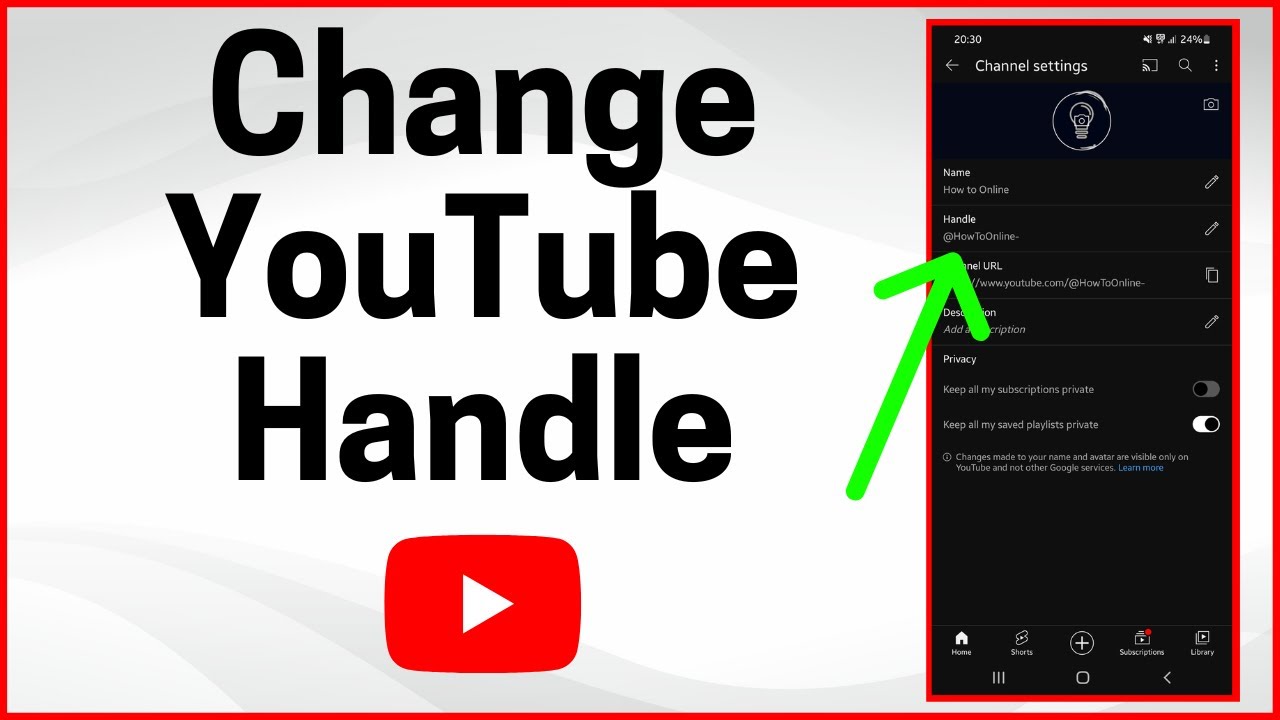This image is a detailed YouTube-themed thumbnail screenshot. The left side of the thumbnail features large, stacked black text on a gray background: "Change" at the top, "YouTube" in the middle, and "Handle" at the bottom. Below "Handle," there is a YouTube logo icon, characterized as a red square with a white play button in the center. The entire thumbnail is framed with a bold red border.

On the right side of the image, there is a screenshot of a smartphone's display, indicating a settings page. A green arrow points upwards towards a section labeled "Handle." The smartphone screenshot is identifiable due to the status bar at the top, which shows the time as 20:30 (8:30 PM), and the battery level at 24%. The top portion of the settings page reads "Channel settings," beneath which appears a light bulb icon encircled by a ring. Below this are various editable fields and options, including "Name," "How to Online," "Handle @howtoonline," "Channel URL," "Description," "Privacy," followed by a checkbox option labeled "Keep all my subscriptions private."